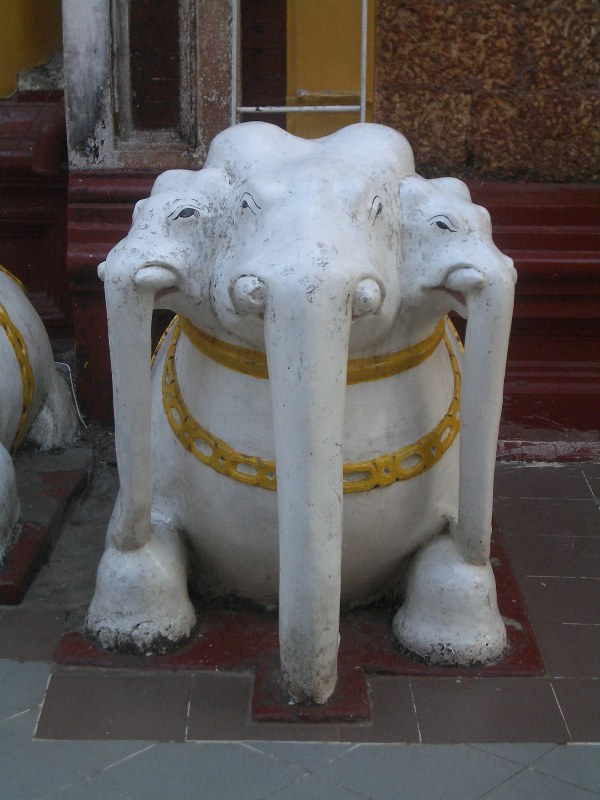The image is a color photograph with either natural or mild indoor lighting, capturing a scene that could be both outside or inside, as it's not entirely clear. The background consists of a gritty city-like building with dark brown molding on the bottom and possibly some plaster or marble texture on the walls. There is an area that appears damaged or is missing a panel, and along the bottom, there might be some layered red molding, though the exact material of the building is uncertain. The ground is tiled with light and dark gray tiles.

In the center stands a prominent, intricate white sculpture, possibly porcelain or stone, featuring a tri-headed elephant design. The sculpture is on a small red pedestal. The central elephant head faces forward with its trunk extending all the way down to the tiled ground. Two smaller elephant heads flank it on either side, with their trunks reaching down to the base of the central figure's feet. All three elephant heads feature very short white tusks and exhibit some texture and signs of wear, accentuated by darker black coloring. Golden ornamental rings adorn the sculpture, one around the neck of the central elephant head and another chain-like design across the body. This detailed and visually striking sculpture seems to hint at a cultural or artistic significance, possibly suggesting a location like India due to its unique design elements. Additionally, a part of a similar statue is visible to the left.